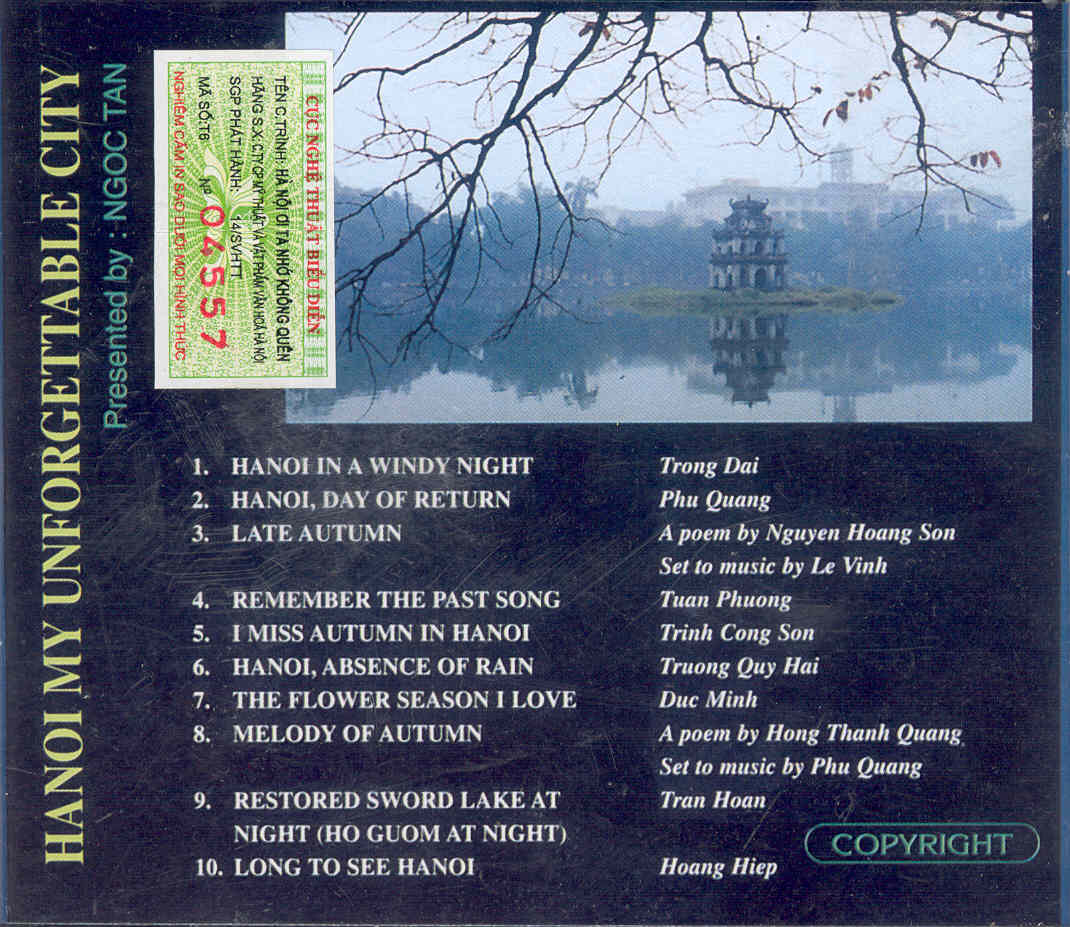The back cover of this CD features a detailed listing of its musical contents against a black background, marred by some visible scratches on the CD case. Dominating the upper portion of the cover is a photograph portraying a serene lake, encircling a small island with a pagoda, and a stately building rising behind bare winter trees. Horizontally to the left, the text reads, “Hanoi, My Unforgettable City,” presented by NGOC10.

The album comprises ten songs, their titles in uppercase and artists’ names in title case, starting with:
1. "Hanoi in a Windy Night" by Trang Dai
2. "Hanoi, Day of Return" by Phu Quang
3. "Late Autumn," a poem by Nguyen Hoang Son, set to music by Le Vinh
4. "Remember the Past Song" by Toan Phuong
5. "I Miss Autumn in Hanoi" by Trinh Cong Son
6. "Hanoi, Absence of Rain" by Truong Quoc Hai
7. "The Flower Season I Love" by Duc Minh
8. "Melody of Autumn," a poem by Hang Thanh Quang, set to music by Phu Quang
9. "Restored Sword Lake at Night" (Ho Guom at Night) by Tran Hoan
10. "Long to See Hanoi" by Hoang Diep

Additionally, there is a green tax stamp with Vietnamese characters, lending an official look, and in the lower right-hand corner, an oval seal containing the word 'copyright' in green writing. This back cover sheet beautifully encapsulates a musical homage to Hanoi.